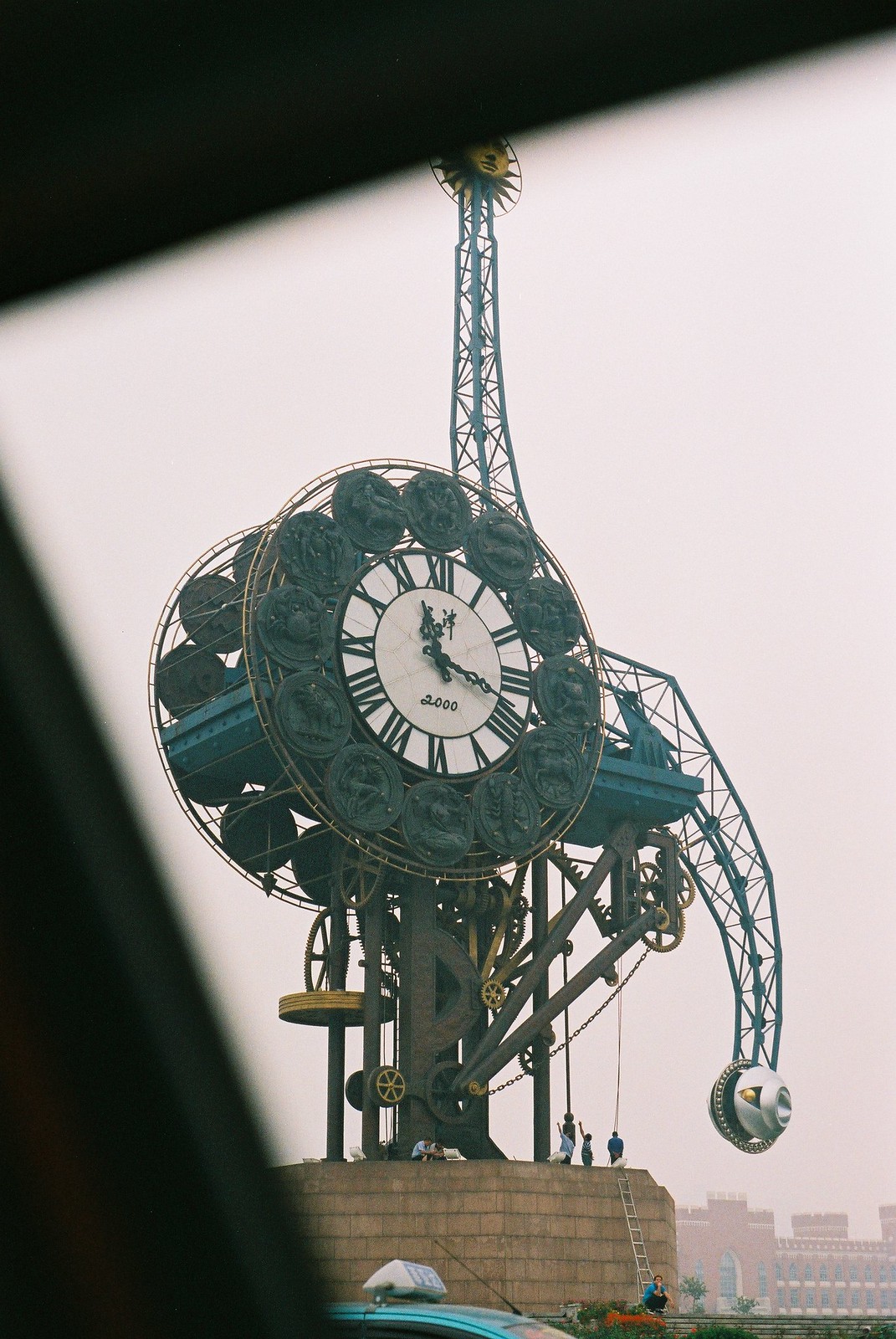The image depicts an elaborate outdoor mechanical clock structure prominently positioned atop a stone building. The clock is supported by multiple metal beams that connect it to the building, and complex gears are visible around the base, extending into a tall ferris wheel-like structure. The clock face features a white background with ornate hands and Roman numerals encircled by images of animals in metal rings. Above the clock face, steel beams extend to support a sun with a face. To the right, an additional beam structure droops downward, ending in what appears to be a bell. Several people are seen standing in front of the clock on top of the building, with a ladder providing access to the right. The top and left diagonal corners of the photograph are black, suggesting it may have been taken from within a car.